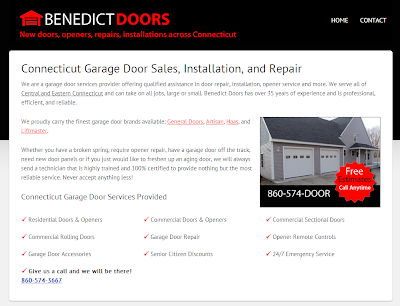A detailed screenshot of the "Benedict Doors" website. At the top-left corner, the website name "Benedict Doors" is prominently displayed, with "Doors" highlighted in red and "Benedict" in white, accompanied by a red icon of a house with a garage door. Below the name, the tagline reads: "New Doors, Openers, Repairs, Installations Across Connecticut."

On the top-right, navigation options "Home" and "Contact" are clearly visible in white text. Centrally at the top, the website highlights its services with the text: "Connecticut Garage, Door Sales, Installation and Repairs."

In the middle-right section, a detailed boxed image of a house with two white garage doors is displayed. Each garage door features four small windowed areas at the top. Below this image, the contact number "860-574-DOOR" is prominently shown, alongside a badge icon stating "Free Estimates. Call anytime."

At the bottom left of the image, the same contact number is repeated in blue text alongside the message: "Give us a call and we will be there."